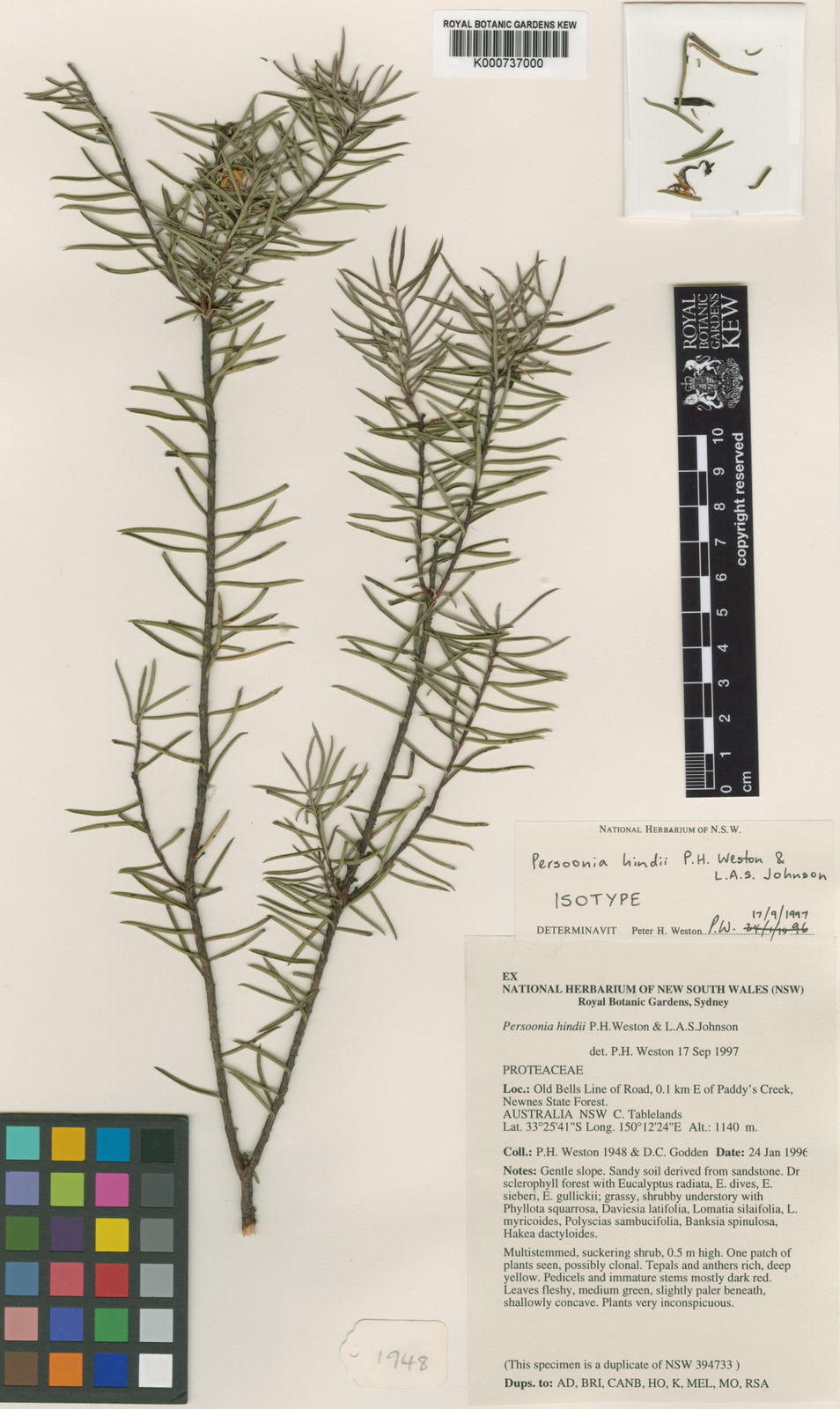The image depicts a beautifully preserved and pressed plant specimen laid out on a piece of paper from the Royal Botanic Gardens, Kew, in England. The detailed exhibit includes a barcode at the top labeled "Royal Botanic Gardens Kew". To the left of the specimen is a ruler marked in centimeters for precise measurement. 

In the top right corner, a few individual shavings of leaves can be seen, suggesting meticulous documentation. At the bottom right corner, there is a detailed description that reads "National Herbarium of NSW, Persunia Hindi, PH, Weston, and LAS Johnson isotype," along with further details like "Determined by Peter H. Weston, PW, 17-9-1997." This text provides both scientific classification and historical context of the specimen. A small tag labeled "1948" rests at the bottom, possibly indicating a significant date related to the plant.

On the bottom left corner, a color palette exhibits a wide range of colors from white through various shades including black, brown, turquoise, blues, pinks, reds, yellows, greens, oranges, purples, and grays, likely serving as a reference for accurate color representation in the documentation of the specimen. The entire setup is displayed against a clean, white background, enhancing the visibility of the plant and accompanying details.